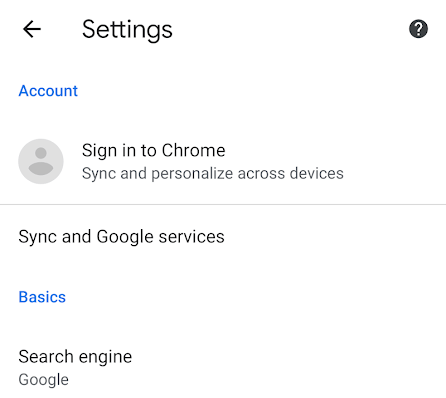This screenshot depicts a settings page for Google Chrome. 

- **Shape and Background:** The image is square in shape and features a clean white background.
  
- **Top Bar:** 
  - In the top left corner, there is a left-facing arrow icon.
  - Right next to the arrow, the word "Settings" is printed in black. 
  - The top right corner hosts a black circle icon with a white question mark in the center, possibly signifying a help or support option.

- **Main Content:** 
  - Directly below the "Settings" heading, on the left side in blue font, it reads "Account."
  - Positioned underneath "Account," there is a gray circle featuring a human figure icon in its center. 
  - To the right of this circle, the text "Sign in to Chrome, sync and personalize across devices" appears in black print.
  
- **Dividing Line:** A thin gray line runs horizontally across the screen, just below the "Sign in to Chrome" section.

- **Subsequent Sections:**
  - Following the horizontal line, "Sync and Google services" is displayed in black text.
  - Beneath this, "Basics" is highlighted in blue font, marking another section.
  - Finally, at the bottom of the page in black font, the text reads "Search engine Google."

This detailed layout helps illustrate the structure and content of the Chrome settings page for better comprehension.